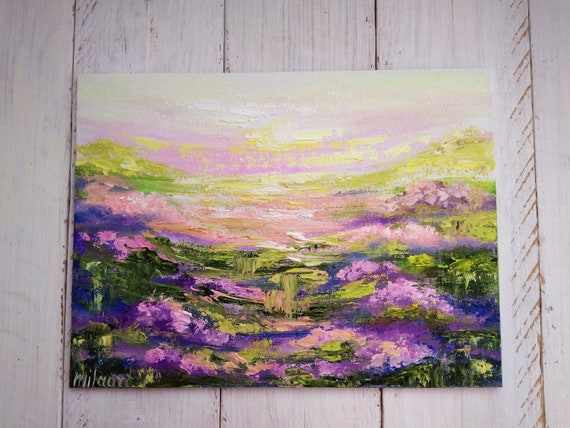This is a photograph of an oil painting mounted against a white wooden wall. The painting, signed "Malari" on the bottom left corner, captures a vivid outdoor scene teeming with nature. Dominated by lush fields and flowering trees, the artwork showcases long green hills stretching under a sky. The scene brims with an array of colors including pastel pinks, purples, greens, as well as hints of blues, yellows, and lavender. At the horizon, a sun or light source peers through the soft cloud formations, illuminating the rich, thick textures of the paint. The lower part of the painting depicts greenery, water, and possibly a swamp or pond, contributing to the painting's vibrant, life-filled atmosphere. This captivating nature landscape, vibrant with life and color, conveys a serene yet lively environment, and is rich with detail.